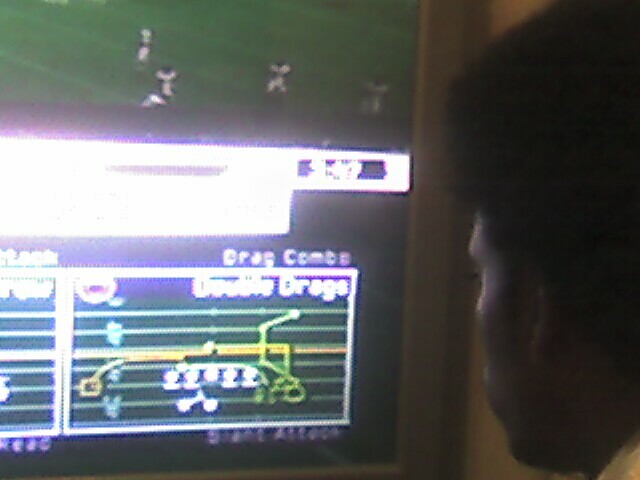This close-up photograph captures a man's side profile as he intently watches a screen, which dominates the left three-quarters of the image. The man, identified by his dark curly afro hair and dark skin, is dressed in what seems to be a lighter-colored shirt visible in the bottom right corner. His gaze is fixed on the screen in front of him, revealing only the outline of his face and a glimpse of his ear.

The screen itself, framed by a couple of inches of a wood border on the right, displays a sports field with visible grass and what appears to be four players. The field is marked with lines typically found in soccer or football. Below this main display is a bright horizontal band of light, separating it from a secondary display.

The lower part of the screen, seemingly a different digital interface, is less discernible but shows the words "drag combo" and "drags." There is also a green rectangle outlined in white with lateral lines, possibly illustrating sports plays or strategies, though the specifics are unclear. Overall, the upper portion resembles a television screen showing live sports, while the lower portion looks like an analytical or informational digital screen.